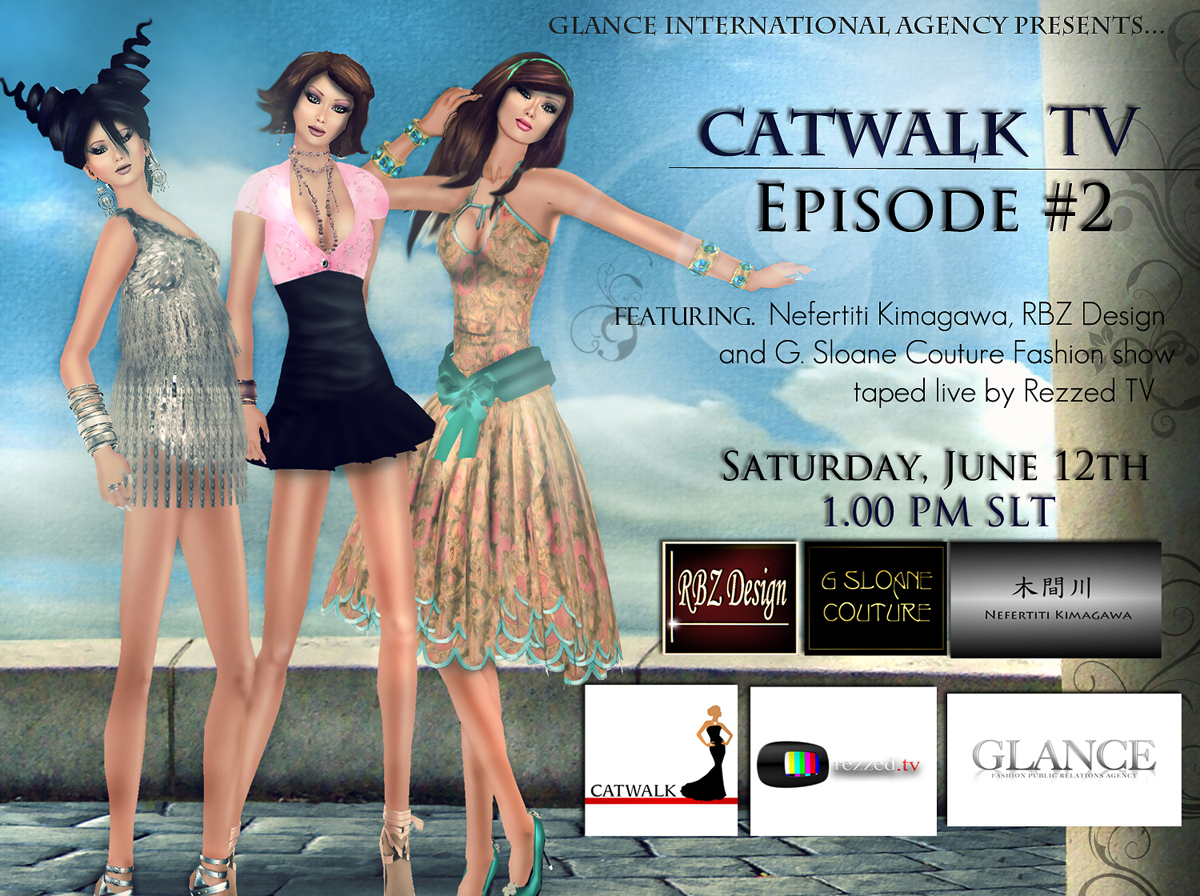The image is a vibrant digital artwork featuring three animated female models standing on a gray cobblestone road next to a gray ledge. The background is predominantly blue with text elements highlighting a fashion show theme. The models, each distinct in their attire and appearance, stand on the left side. The leftmost model sports creative hair, long earrings, numerous bracelets, and a silver dress. The middle model, who appears exceptionally tall, wears a stylish one-piece outfit with a pink top and black skirt. The rightmost model dons a long yellow dress with blue trim, a blue belt, and green heels. Above them, the text reads “Catwalk TV Episode Number Two” in black letters. 

In the bottom right of the image, a collection of square icons is displayed. These icons include “catwalk” on a white background with a red line and a woman in a black dress, and the logo "resd.tv" in white and red on a black screen featuring various colors like white, yellow, green, purple, red, and blue. Other sponsors and contributors are listed, such as “G Sloan Korcher” in yellow on a black background, "RBZ Design" in white on black, and “Nifredi Kinagawa” in black on gray. 

Additional details include Chinese characters in black and various other texts like “Glance” on a white background. The event is highlighted to air on “Saturday, June 12th, 1:00 p.m. SLT” with the main feature being the fashion show "taped live by resd.tv," emphasizing contributions from Nifredi Kinagawa, RBZ Design, and G Sloan Korcher.